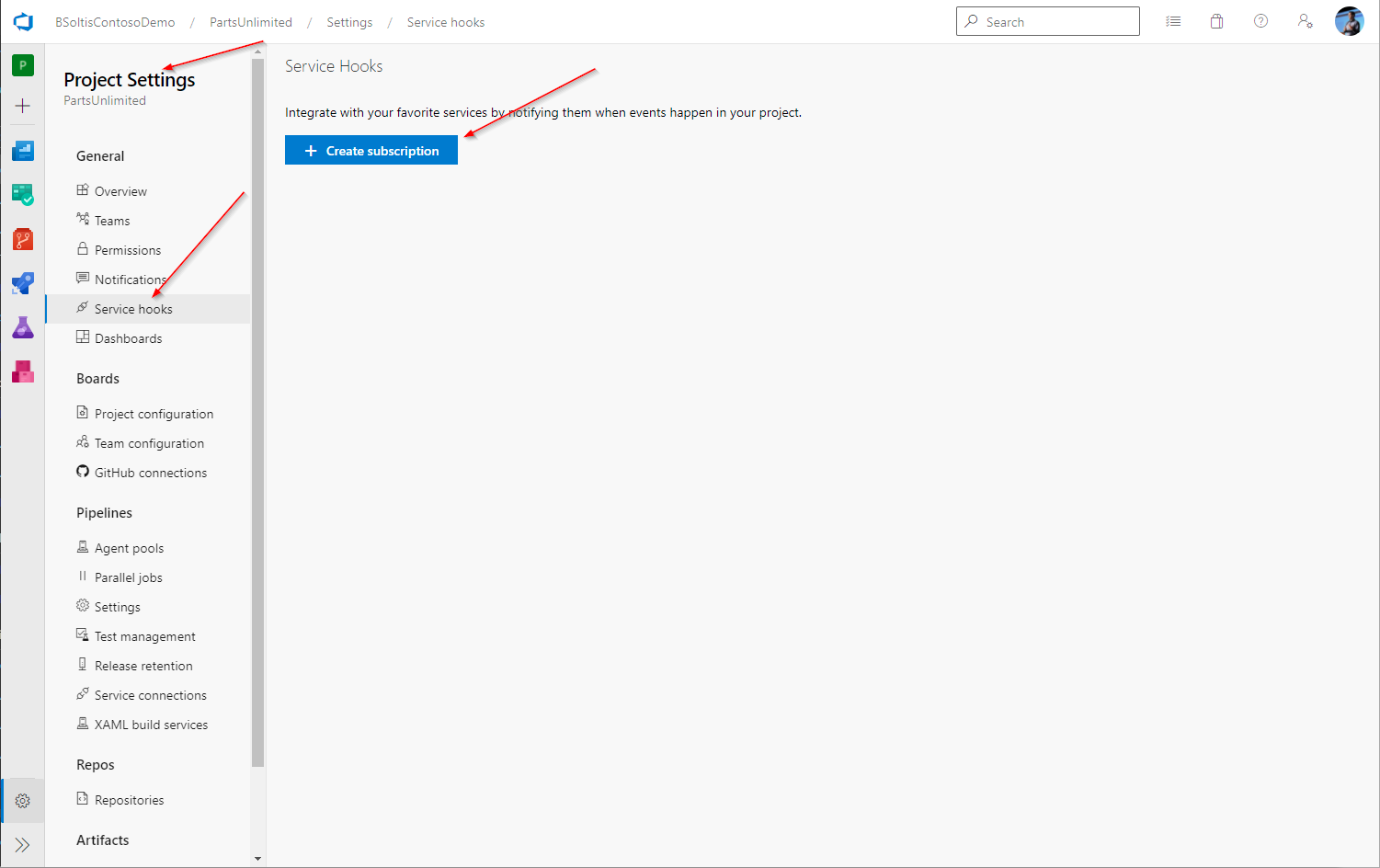A detailed and cleaned-up caption for the image:

"The computer screen displays the Project Settings page on a Windows PC. On the left sidebar, Project Settings is highlighted and indicated by a red arrow. The subheadings under Project Settings include General, Boards, Pipelines, Repos, and Artifacts. Within the General section, Service Hooks is emphasized with another red arrow. Service Hooks occupies the majority of the page, describing its function as a tool to integrate with favorite services by notifying them of project events. A third red arrow points to 'Create Subscription,' prominently positioned for user action. The top right corner features a search icon, battery indicator, help icon, and a partially visible user profile picture."